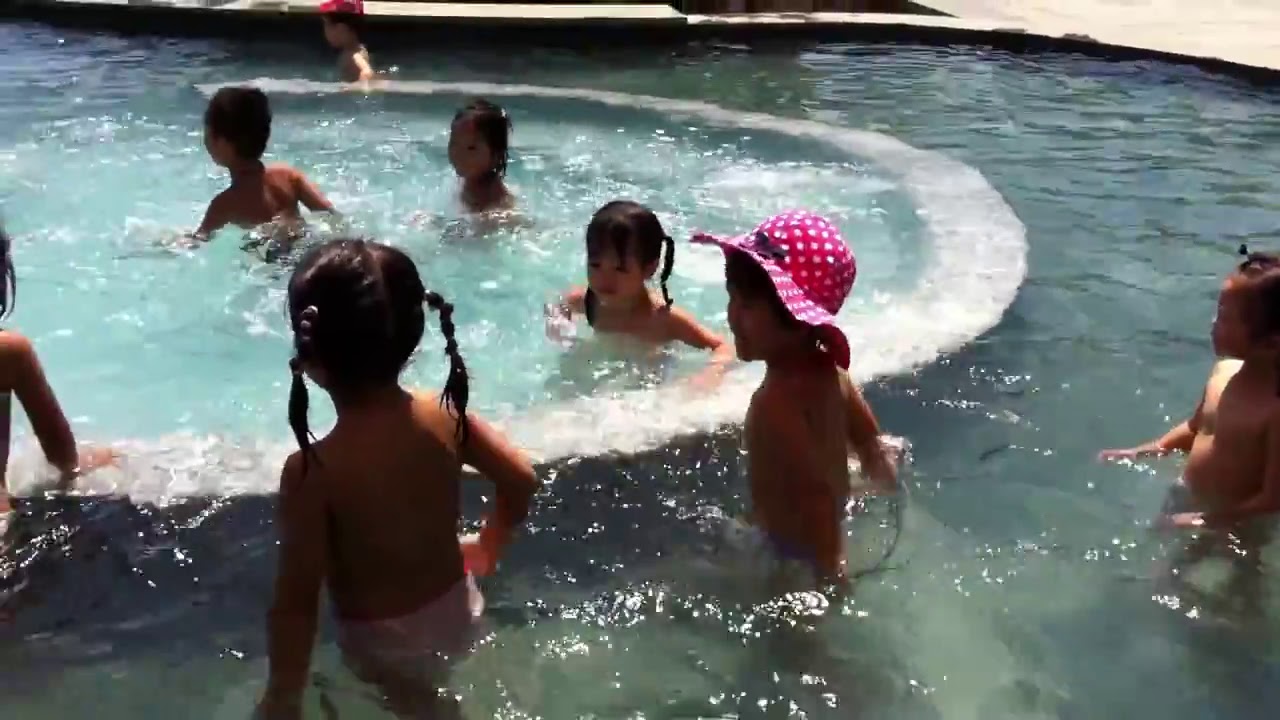In this vivid and dynamic outdoor scene, captured on a sunny day, a group of eight children are joyfully playing in a large public swimming pool. The pool, with its inviting clear water that transitions from light to dark blue, features a central white circular structure, likely a set of steps leading to the deeper section. The pool's backdrop includes stone pavement, hinting at its public setting. The children are clothed in various colorful swimwear, with one noticeable detail being a girl wearing a pink hat adorned with red polka dots and a tiny bow. Another distinctive feature includes two girls sporting pigtails. The water is alive with their playful splashing, which glistens in the bright sunlight, enhancing the overall jubilant atmosphere of a summer day.